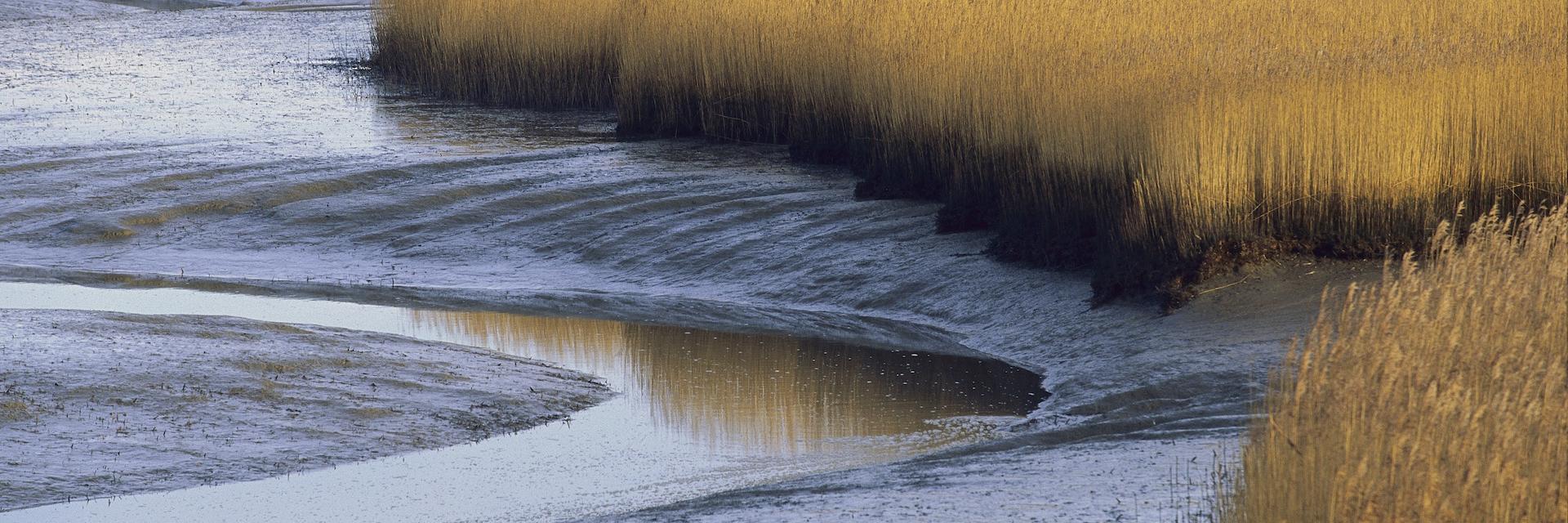In the photograph, a serpentine river begins at the bottom left and winds towards the center before curving back sharply, forming a sideways U-shape. It then flows towards the right side of the image and exits the frame. The river is bordered by wet, dark brown soil. To the far right, behind the river, a dense cluster of tall reeds stands. The reeds exhibit a gradient in color: dark brown at the base where they meet the soil, transitioning to a golden hay color as they extend upward, possibly indicating the fall season. These reeds dominate the right side of the photograph, with some appearing to emerge directly from the water. Meanwhile, on the left side, the river reflects some of the reeds, adding to the serene, aquatic ambiance of the scene.